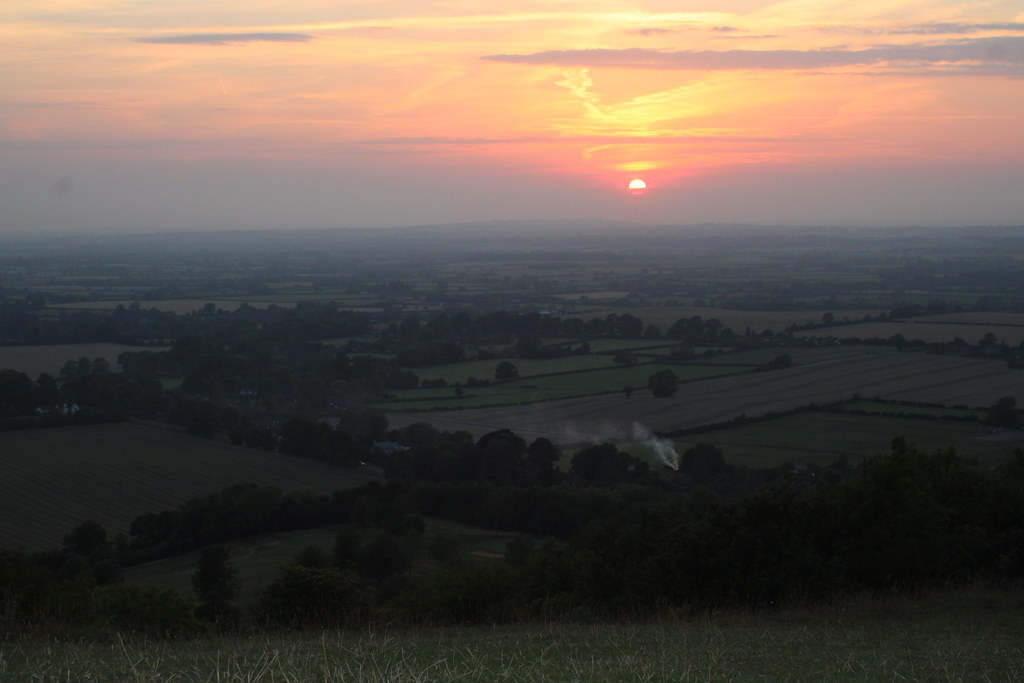This is a landscape photograph capturing an expansive valley during a sunset or possibly sunrise. The bottom half of the image is dark, revealing rolling hills and vast open fields of greenery, dotted with trees and vegetation, stretching into the distance. In the foreground, a slope covered in lush green grasses is visible. The top half of the photo showcases a dramatic sky where hues of yellow, orange, and pink blend seamlessly into grays, indicative of a cloudy day. The very top of the image features a bright half-moon, which contrasts starkly against the colorful sky. This peaceful scene also includes mist covering the distant end of the valley, adding to the tranquil ambiance. The photograph is devoid of text, people, or any urban elements, emphasizing the serene beauty of nature.